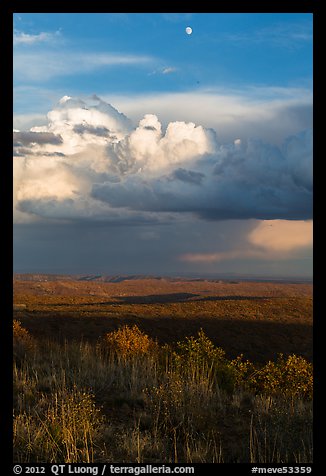The photograph framed by a black border, with the watermark "© 2012 QT Luong, TerraGalleria.com #Meve53359," showcases a nature scene predominantly composed of sky and land. Over half of the image's upper portion is dominated by a blue sky featuring a partially visible moon and a variety of clouds. At the top, the sky is a rich blue transitioning to a grayer, darker hue toward the bottom. A large, dense row of clouds stretches across the sky, appearing white and turning darker and murkier toward the horizon. Below the sky lay a sprawling brownish prairie devoid of animals, appearing relatively barren except for patches of green and hay-colored plants near the bottom. The fields extend towards distant, shadowed mountains, enhancing a sense of vast, untouched wilderness.